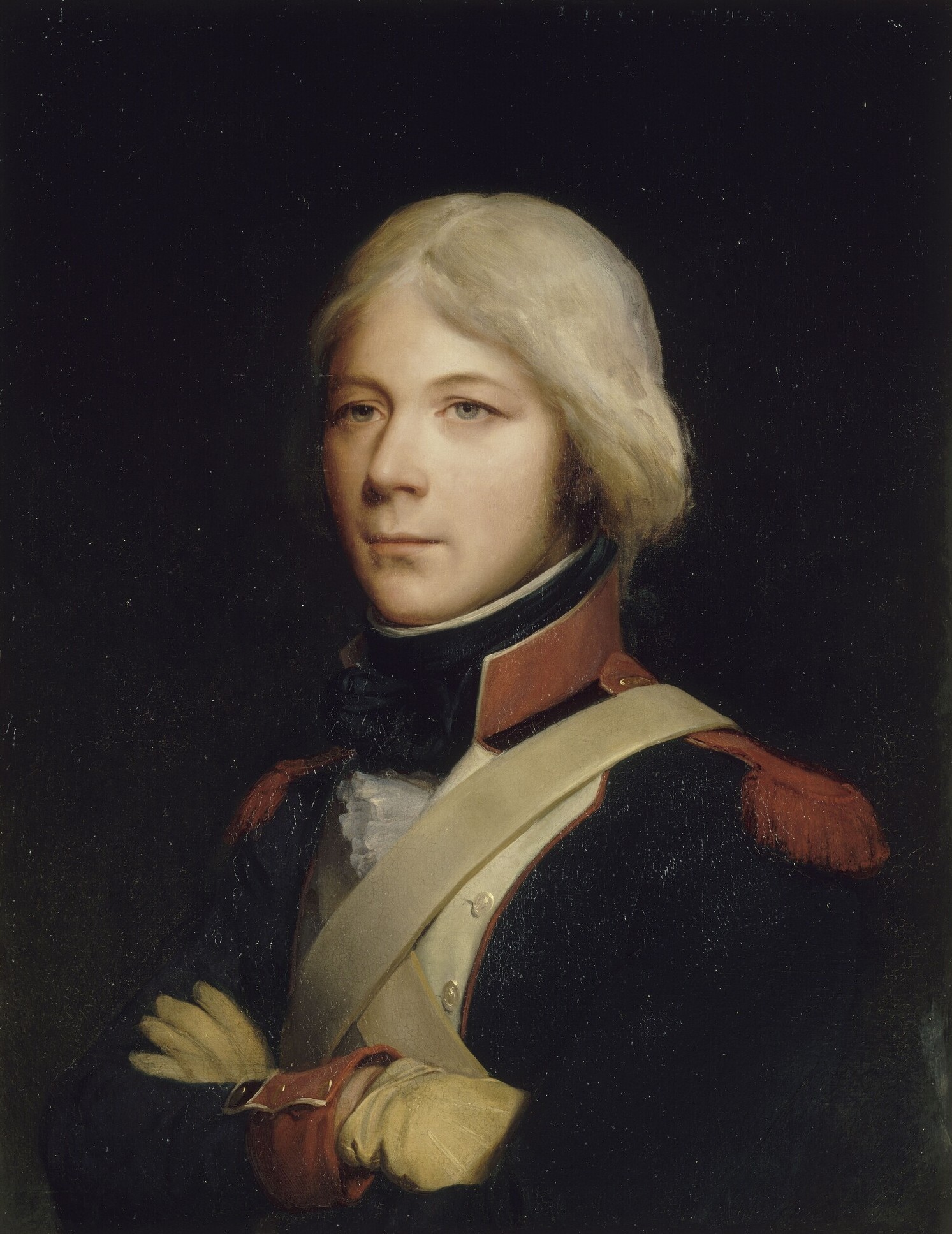The image is a detailed portrait of a very young man, possibly in his late teens or early twenties, depicted in a military-style uniform. His light-colored hair, appearing either blonde or silver, is styled in a low ponytail. His light-colored eyes, either green or blue, are framed by a determined expression with pursed lips, while he looks slightly away from the viewer. He has a light complexion, and his arms are crossed in front of him, covered in tan gloves.

His attire is intricate and formal, consisting of a dark blue or black overcoat adorned with red fringes on the shoulders and a red collar. The cuffs of the sleeves are also red. A sash runs diagonally from his left shoulder down to his right side. Underneath the overcoat, he wears a shirt with elaborate white frills and black frills at the neck, complemented by a blue collar. The portrait's background is black, focusing all attention on the singular, central figure with no additional writing or elements visible.